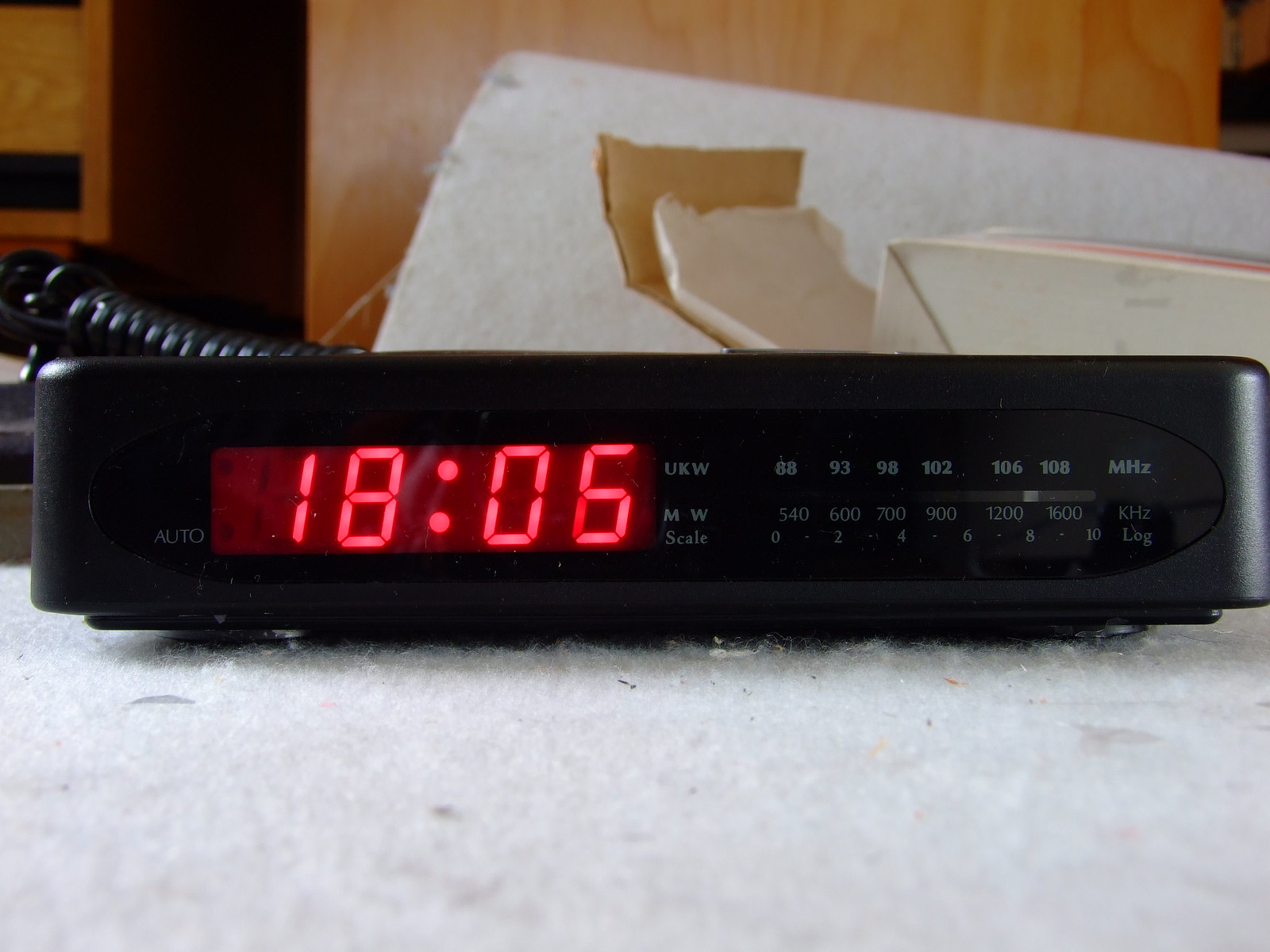The image shows a scene with various elements. At the top end, there is a wooden wall with a light finish. Draped over this wall and cascading down to the ground is some white felt fabric. Near the bottom of the wall, there is a piece of brown cardboard and to the right of it sits a white box with a fold at the bottom.

On the left side of the scene, there is a coiled cable, likely a phone cable, attached to what seems to be a clock. This clock features a predominantly black ring. The display on the clock reads "18:06" in red digits. Below the time, the word "Auto" is written. In the top right corner of the clock, "UKW" is displayed, and just underneath it, there are the letters "MW" followed by the word "scale." The clock also has a frequency scale with markings: 88, 93, 98, 102, 106, and 108 megahertz on the FM band, and 540, 600, 700, 900, 1200, 1600 kilohertz on the AM band. Additionally, a logarithmic scale with markings at 0, 2, 4, 6, 8, and 10 is present at the bottom of the display.